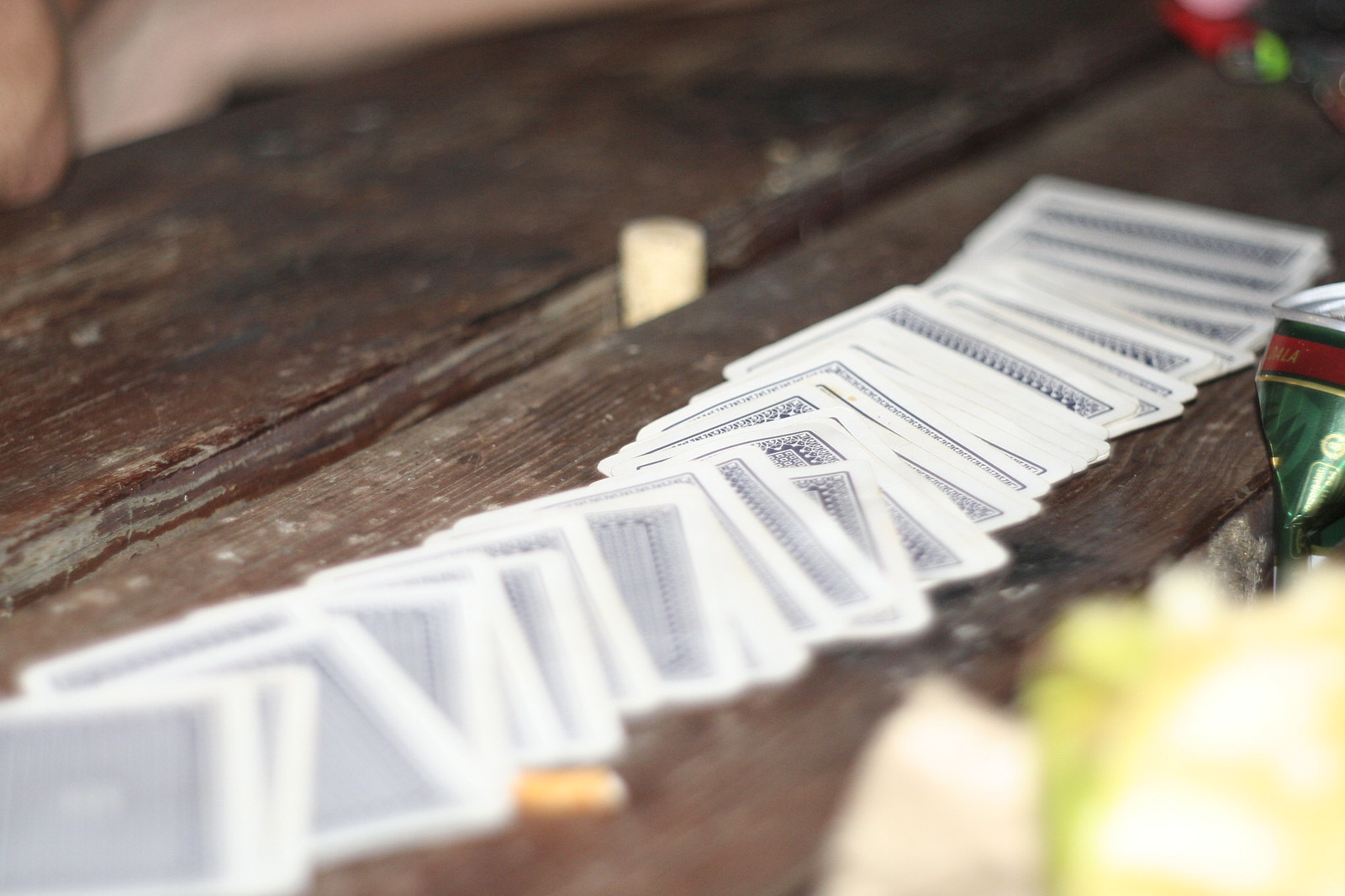The image displays a top-down view of a table. Scattered across the surface are various playing cards, each outlined in white with blue and black designs on the back. Prominently centered amidst the cards is what appears to be a ticket. In the bottom right corner, there is a green beverage, with small green objects or fragments nearby. The table itself has a brown background, adding a warm and rustic touch to the setting.